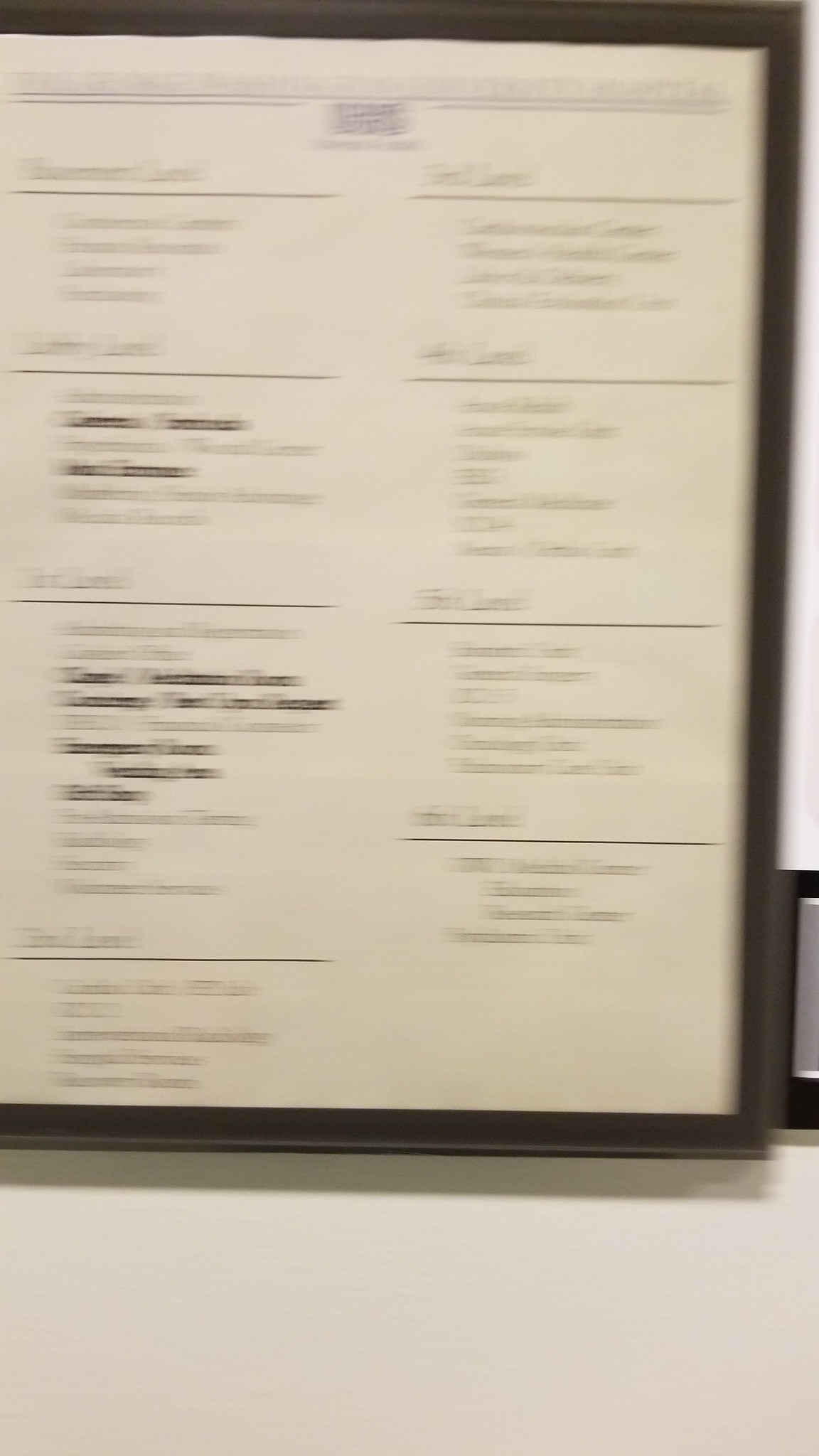The image depicts a very blurry photograph of a white piece of paper surrounded by a dark, possibly wooden frame, or it could be a gray clipboard. The paper features a mix of black and gray text, with some sections in bold for emphasis. The text is mostly unreadable due to the blurriness, but it appears to be organized into different categories or headers, possibly resembling a worksheet or a menu with two columns of divided information. There is a logo at the top that seems to be in black and blue. The frame casts a shadow on a white wall behind it. The layout of the text suggests an organized format with headers and sub-sections, but specific details remain indiscernible.